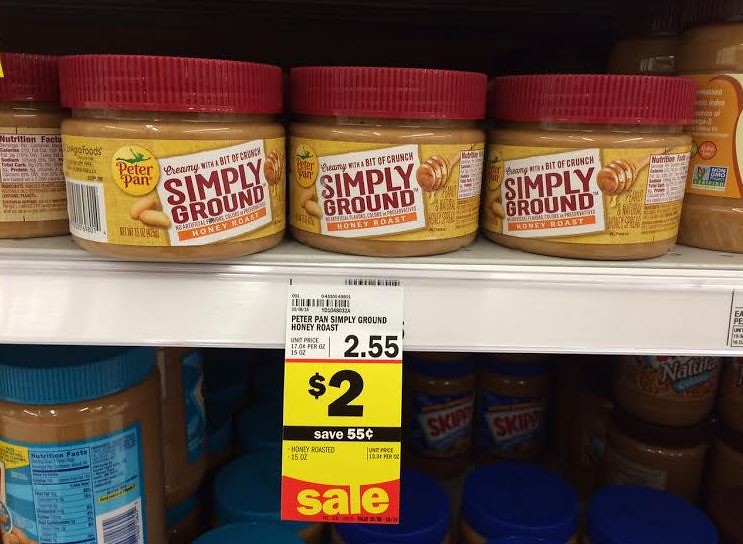The photograph appears to be taken inside a grocery store, focusing closely on a shelf stocked with various jars of peanut butter. On the top shelf, there are smaller plastic jars of Peter Pan Simply Ground Honey Roast Peanut Butter, identifiable by their burgundy lids. The labels on these jars indicate "Peter Pan Creamy with a Bit of Crunch Simply Ground" and "Honey Roast."

Below these jars, a price tag displays the regular price of $2.55. An additional, more prominent yellow tag underneath announces a sale, stating "$2.00" with a note of "Save 55 cents," highlighting that the peanut butter is currently discounted.

In the lower part of the image, another shelf is partially visible, stocked with Skippy peanut butter jars, distinguishable by their blue lids. However, this section is dimly lit and less focused, drawing less attention compared to the prominently displayed sale on the Peter Pan Simply Ground Honey Roast peanut butter. The primary focus of the photograph is evidently the discounted Peter Pan product on the top shelf.